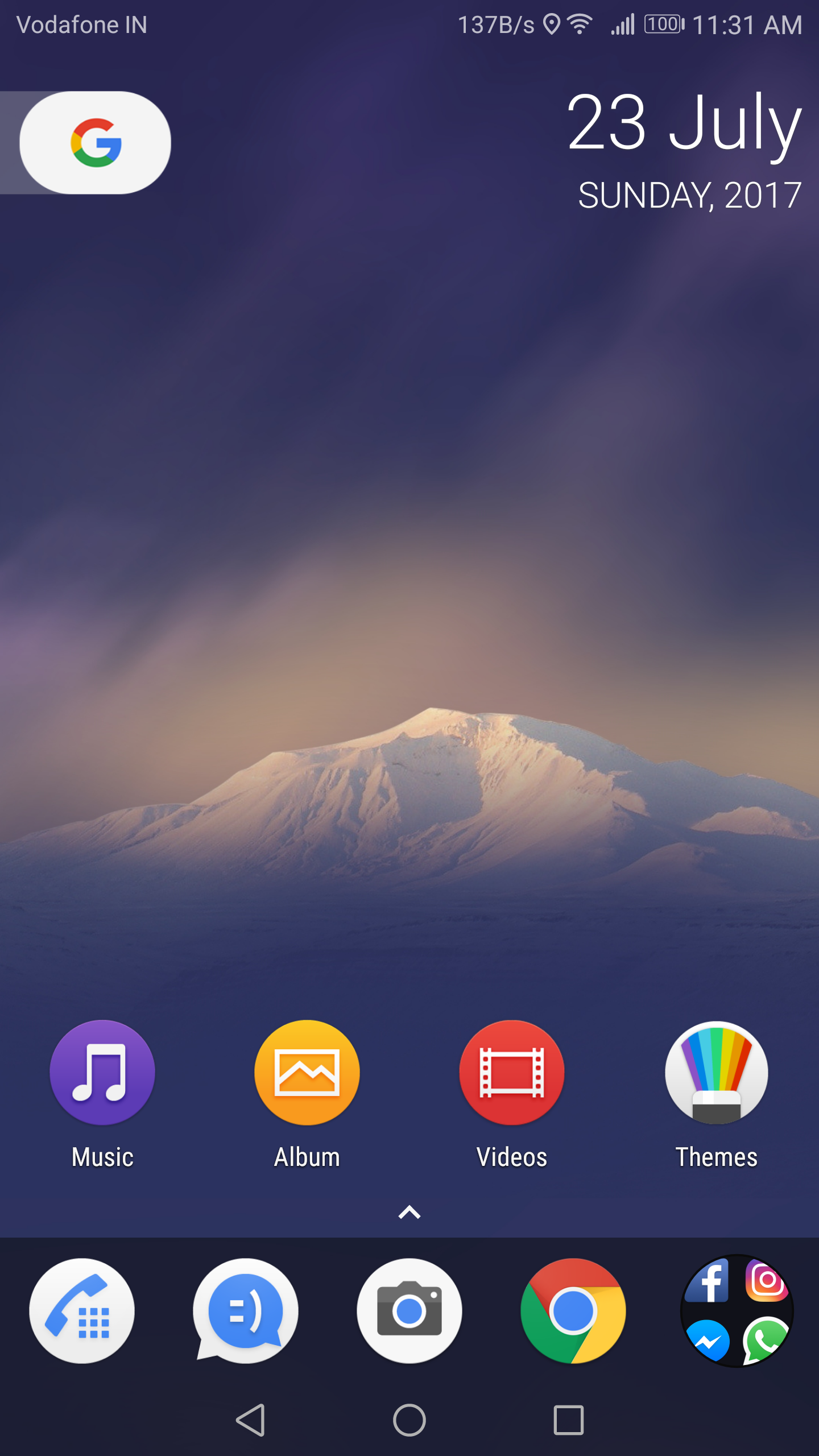The image showcases a Vodafone AIN mobile interface with full WiFi signal and battery status at 100%. The time displayed is 11:31 AM on Sunday, July 23, 2017. At the top of the screen, there is a black section followed by a white area, transitioning into a picturesque scene of snow-peaked mountains with dark shadows cast over the snow, contrasting against a clear blue sky.

The interface contains several options: 
- "Music" in blue
- "Album" in orange
- "Videos" in red

There are also themes displayed, including a rainbow theme. A yellow-white circular icon is labeled "Phone." Additional icons shown are:
- Smiley face
- Camera
- Google Chrome in red, yellow, green, and blue
- Facebook
- Instagram
- Facebook Messenger
- WhatsApp

At the bottom of the screen, a black bar contains buttons with symbols: a sideways triangle, a circle, and a square, typically representing navigation buttons on a mobile device.

This appears to be a nature-themed mobile wallpaper or background, emphasizing the snow-capped mountains and the various app icons available on the screen.